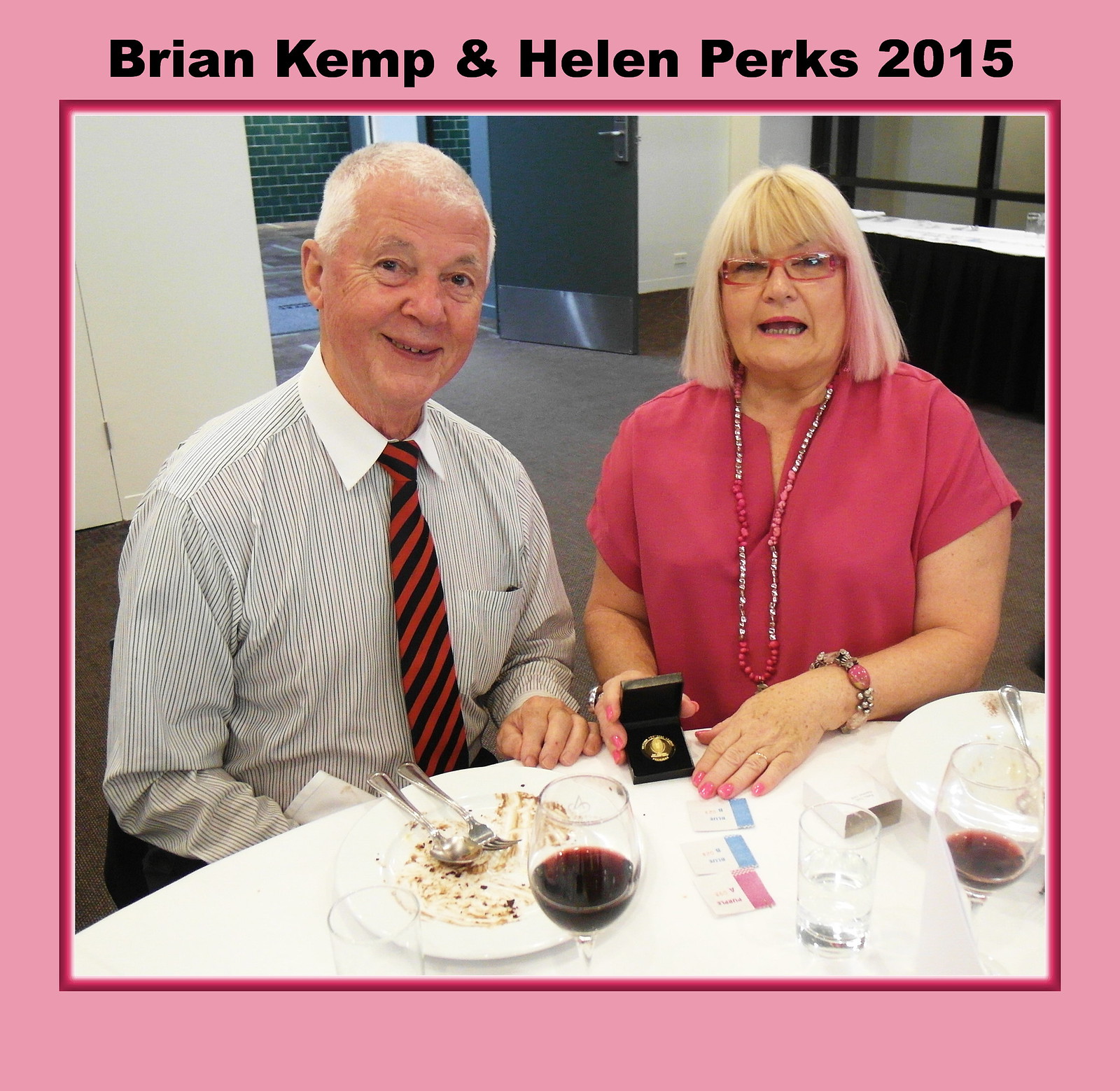The image depicts an elderly couple, likely in their 60s or 70s, seated at a table covered with empty plates and some slips of paper. The man, positioned on the left, has short gray hair and is smiling at the camera. He wears a white dress shirt with stripes, paired with a blue and red striped tie. The woman, seated on the right, has shoulder-length platinum blonde hair and wears glasses. She is dressed in a pink top and a long necklace, with a bracelet on her left wrist and pink-painted fingernails. Her right hand is holding an open box that appears to contain a gold coin or badge. The table also has another box and some cards with pink and blue bars on them. The room has gray carpeting and white walls, with an open door revealing a brick-walled hallway. At the top of the image, black text reads "Brian Kemp & Helen Perks, 2015," and the picture is framed by a pink border.